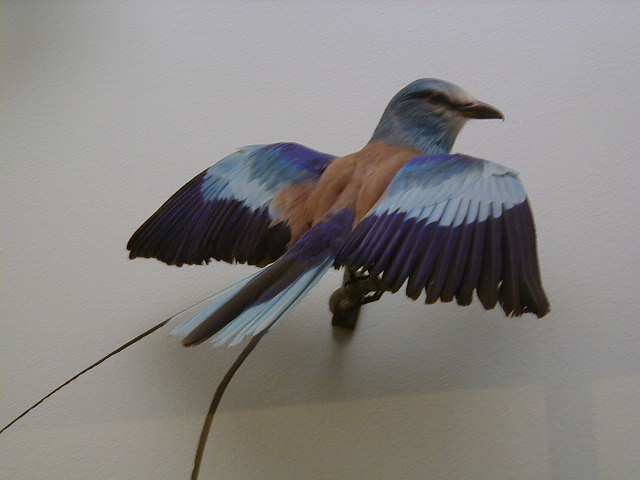The photo depicts a bird mounted on a white or pale blue wall, giving the impression of a taxidermy display or a high-quality painting. The bird appears incredibly lifelike, despite the artificial setting. Its wings are fully outstretched, showcasing a gradient of colors. The upper parts of the wings are dark blue or black fading into various shades of lighter blue and white towards the tips, with darker hues at the edges. The bird’s body is primarily a light brownish-orange, and its head, turned to the right, is light blue with white accents. The back of the bird exhibits an orangish tone, transitioning into purple and blue feathers near the tail. The tail itself features a mix of brown, light blue, and white tips, along with two long brown feathers extending outward. The bird's feet are clasped onto a brass or wooden piece protruding from the wall, adding to the display’s realism. The overall dimensions of the image suggest it is rectangular, about four inches tall and five inches wide.